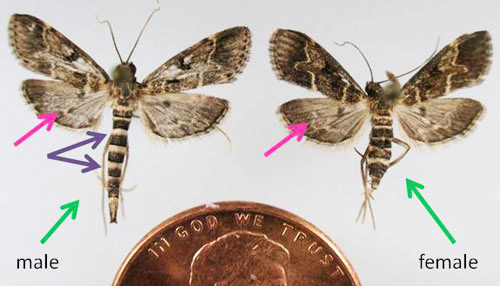This image is a detailed diagram depicting two butterflies, one male on the left and one female on the right, against a light blue-gray backdrop. Each butterfly's distinguishing features are identified with various colored arrows. Pink arrows point to their wings, while purple arrows indicate different aspects of their bodies. Green arrows specifically denote the male and female butterflies. For scale, there is a partial image of a copper penny showing the top with "In God We Trust" and the head of Abraham Lincoln, emphasizing the relative size of the butterflies. The butterflies have brown and white coloration with characteristic rings on their tails, which help in their identification as male and female.